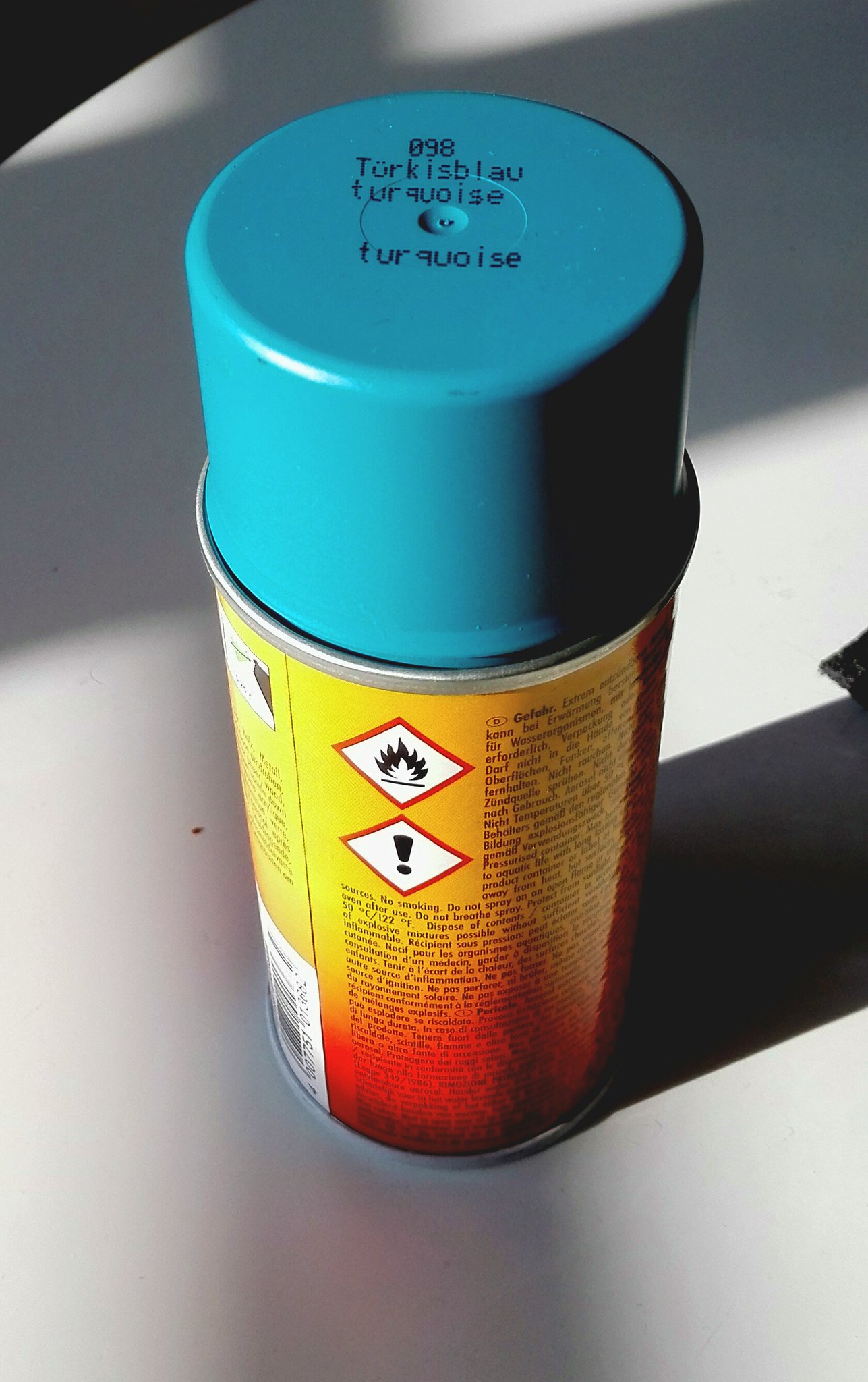The image is a vertically aligned rectangle featuring a close-up of a can of spray paint. The can occupies most of the frame and is seated on a white surface which shows several shadows, including a noticeable rectangular one, as well as a small speck or piece of dirt to the left of the can. In the upper left corner of the image, there is a triangular area of solid black. The spray can itself has a circular, cylindrical body with a prominent turquoise blue cap. On the top of the cap, "098 turquoise blue turquoise" is printed in black text. The body of the can is primarily yellow with shading of red near the bottom, and it includes various instructions or cautionary information that are too small to decipher. Two diamond-shaped warning symbols with red borders are visible towards the top of the yellow label, displaying icons for fire hazard and general caution (exclamation mark). Additionally, there is a vertically aligned UPC label from the table surface upward toward the cap.